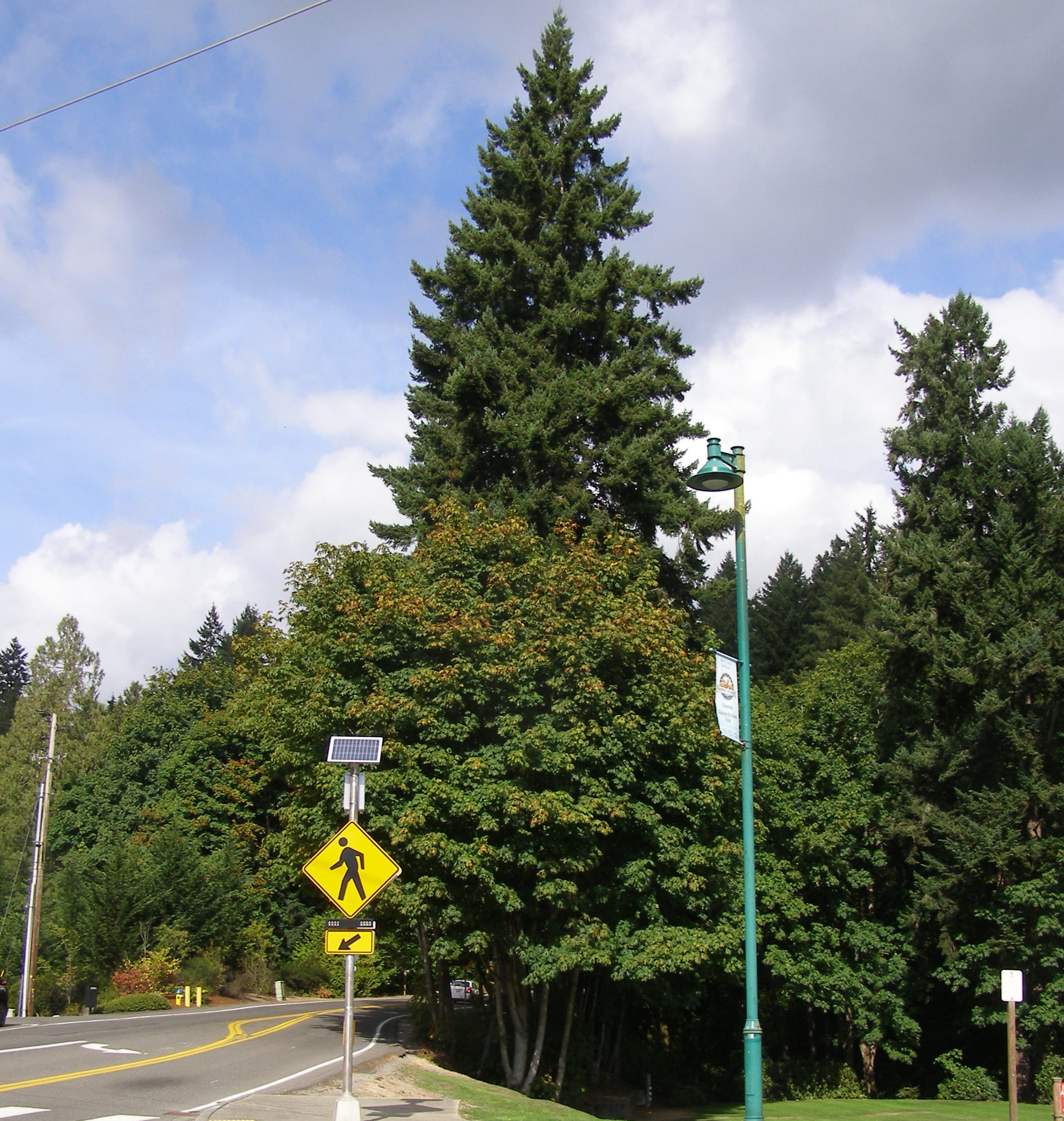This photo captures a sunny outdoor scene with a well-maintained street coming from the bottom left corner and extending upwards. To the right of the street, a pedestrian crosswalk is marked by a triangular sign featuring a walking figure; it has a solar panel on top. A stylish, tall light green lamppost stands nearby, adorned with an unreadable small banner. The right side of the photo showcases a grassy area and towering trees, including pines and some deciduous trees displaying green, yellow, and orange foliage, indicating a colder climate. The background reveals a mix of tall trees and partial clouds, contributing to the bright, natural light illuminating the scene.